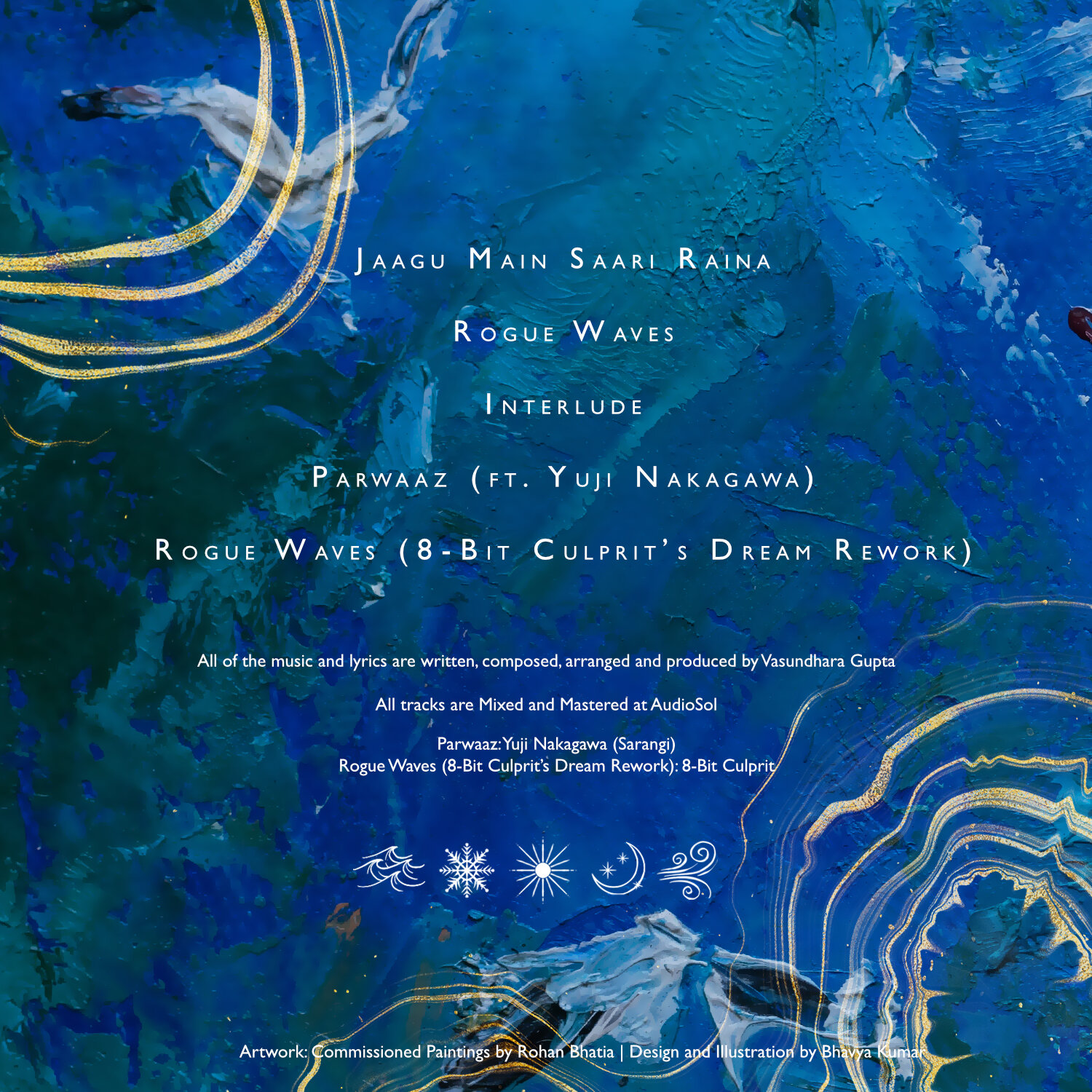The image depicts the back cover of an album, predominantly featuring a blue background with varying shades and abstract designs. Accents of white, black, and gold stripes are present, particularly at the top left and bottom right corners. The text on the image lists the track titles in the following order: "Jagu Main Sari Raina," "Rogue Waves," "Interlude," "Parwaz" (featuring Yuji Nakagawa), and "Rogue Waves (8-Bit Culprit's Dream Rework)." Additional details reveal that all music and lyrics have been written, composed, arranged, and produced by Vasundhara Gupta, with mixing and mastering done at Audio Soul.

The artwork also mentions that "Parwaz" features Yuji Nakagawa on Sarangi and includes visual elements such as icons for waves, a snowflake, the sun, the moon, and wind. The cover boasts commissioned paintings by Rohan Bhatia, with design and illustrations by Bhavya Kumar. The overall aesthetic is abstract with a blue-dominant color scheme, highlighted by sporadic gold elements.